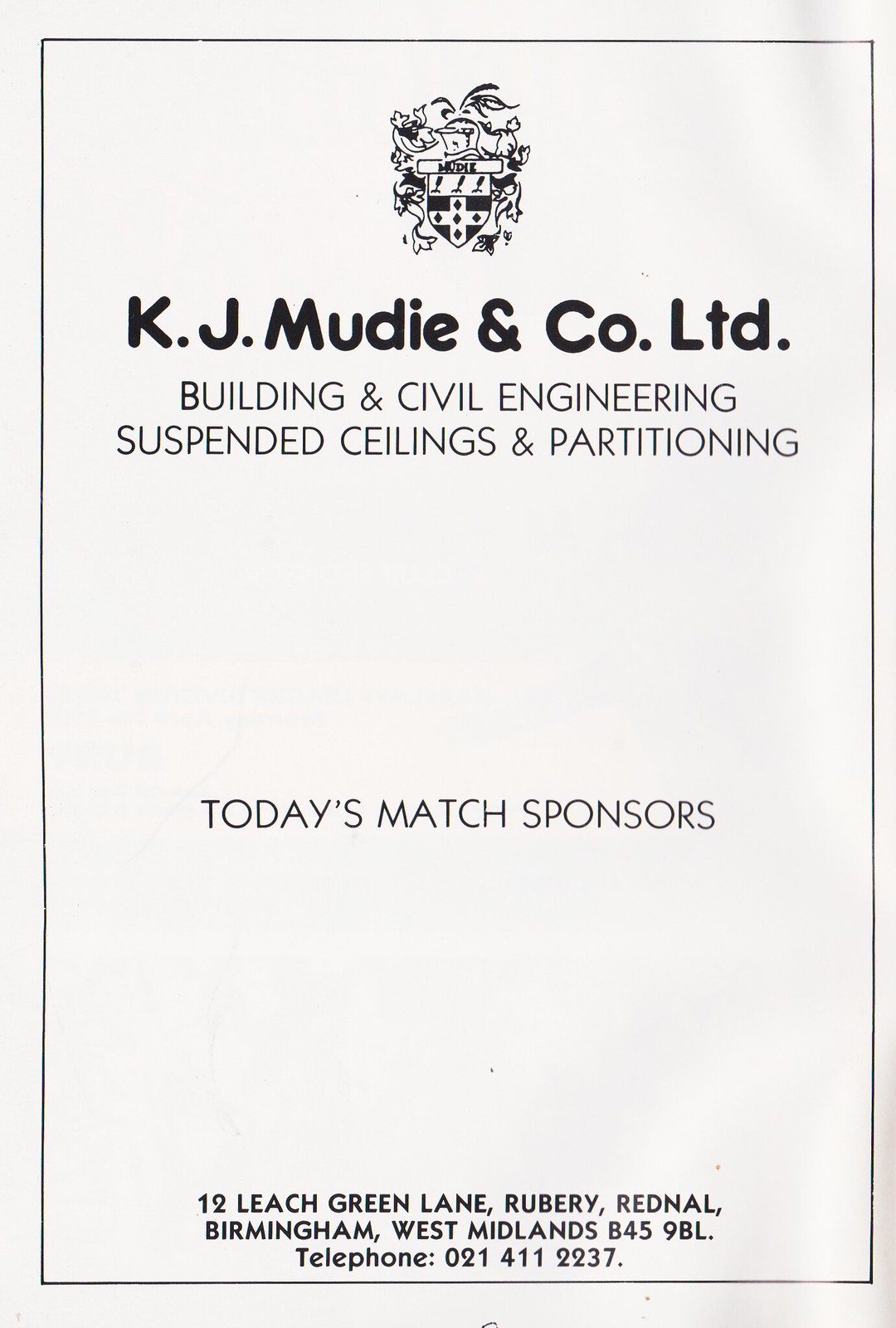The image features a stark white background with black text and includes a small logo centered at the top. Below the logo, the text prominently displays "KJ Muddy and Company LTD." Subsequent lines read "Building and Civil Engineering," "Suspended Ceilings and Partitioning," and "Today's Match Sponsors." At the bottom of the page, an address is listed: "12 Leach Green Lane, Rubery, Rednal, Birmingham, West Midlands, B45 9BL," followed by a telephone number "021-411-2237." The overall design is simple and resembles a magazine cover or program page, indicating sponsorship for an event.